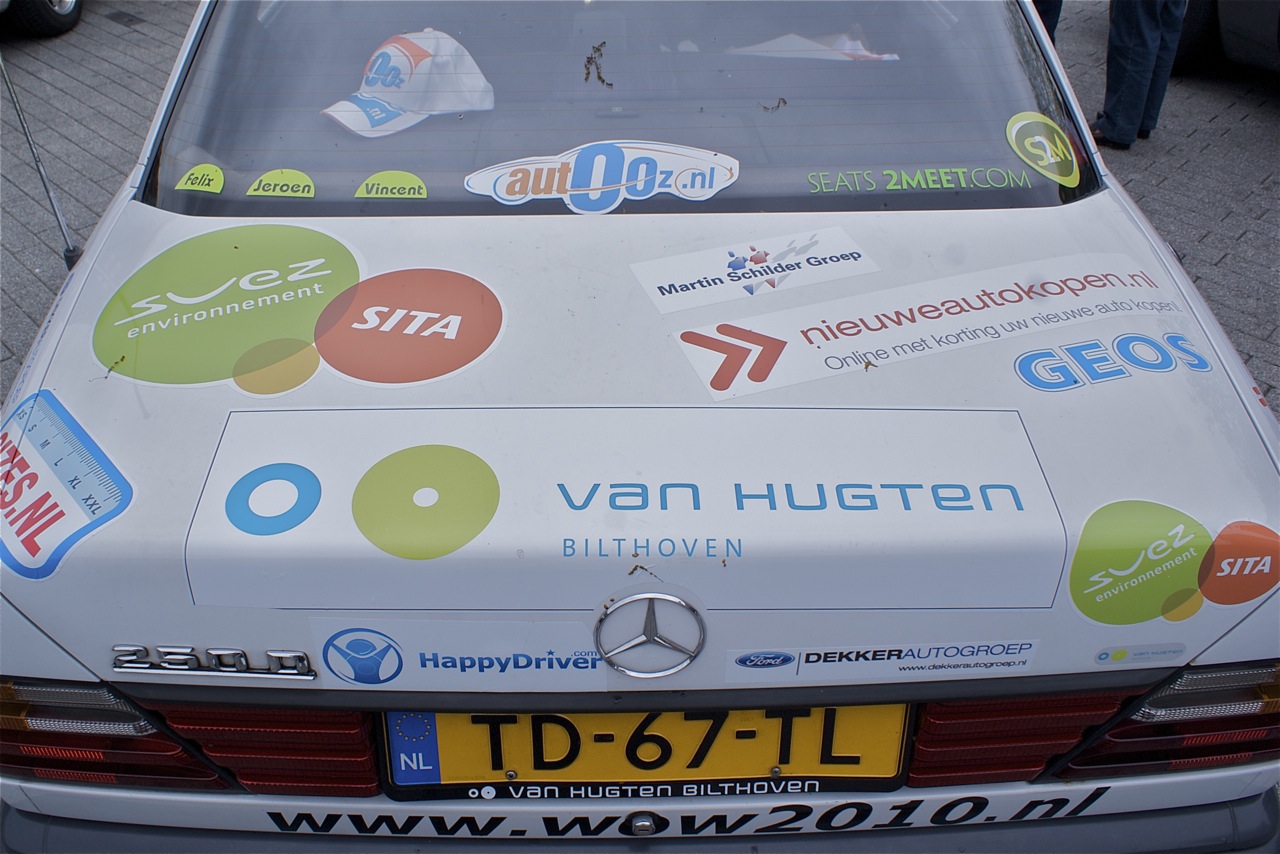In this close-up image of the rear of a white, older-model Mercedes-Benz 2500, which appears to be used for advertising, the trunk is covered with various stickers. Prominent among them are a green circular sticker and a smaller red circular sticker with "SITA" in white lettering. Additional stickers include those with blue lettering reading "Van Huntsman" and "Bilthoven." The bumper displays the web address "www.wow2010.nl" beneath an orange license plate with the number "TD67TL" in raised black lettering.

Through the rear windshield, which also features stickers, a white rally cap with blue text inside the car is visible. Surrounding the vehicle, grey paved stones or a concrete pad can be seen beneath a partially visible wheel on the left and the legs of a person wearing dark blue formal pants and dark shoes on the right.